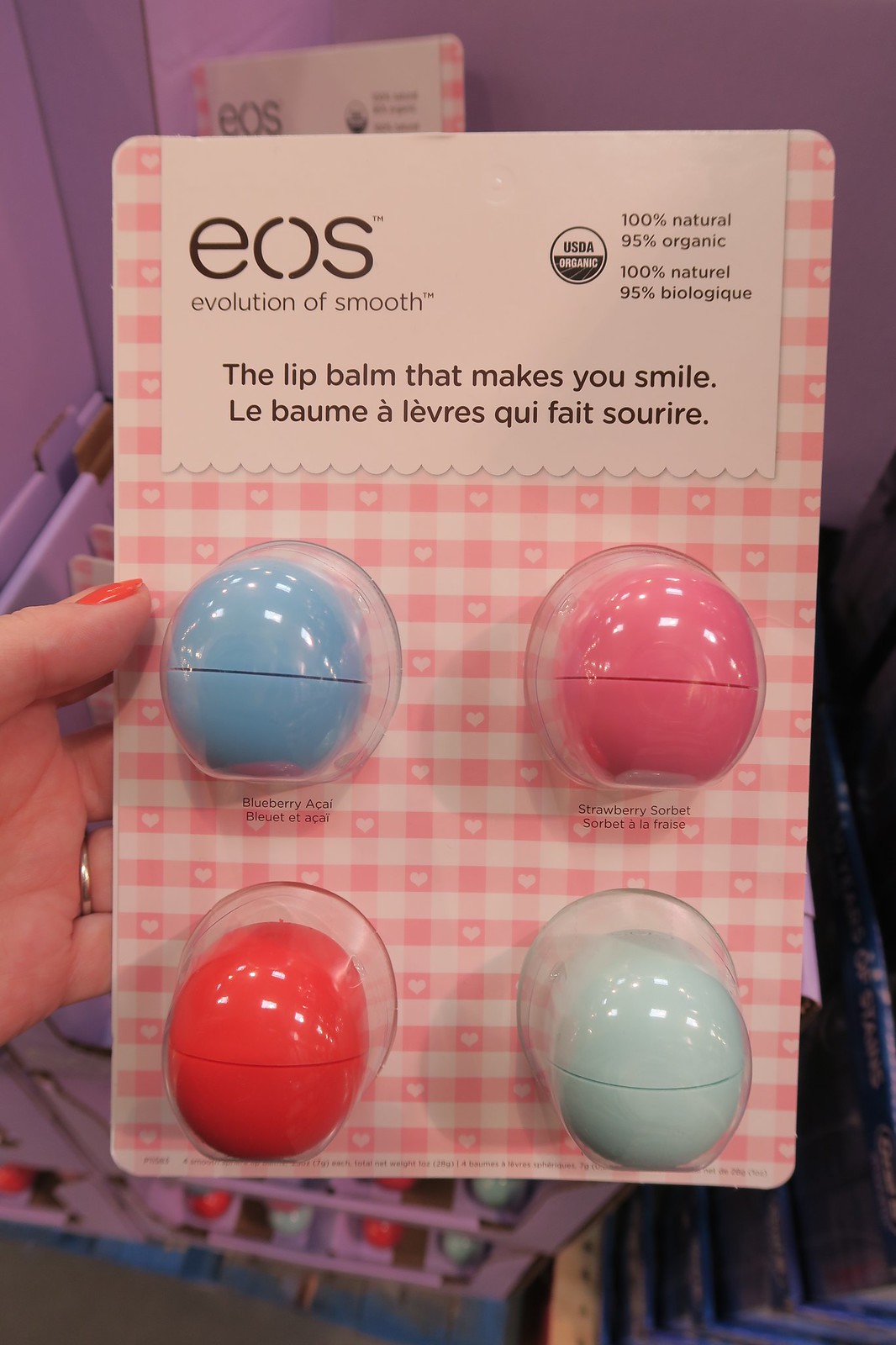In this photograph, a woman's hand adorned with a simple gold ring on her ring finger and bright red nail polish on her thumb is holding up a package of EOS (Evolution of Smooth) lip balms. The package features a pink and white checkered pattern resembling a tablecloth, with some of the dark pink squares containing white hearts. Prominently displayed at the top of the package, in both English and French, are the words "EOS Evolution of Smooth," "100% natural, 95% organic," "100% naturel, 95% biologique," and "The lip balm that makes you smile," "Le Baume à lèvres qui fait sourire." The package contains four egg-shaped lip balms encased in clear plastic pods arranged in a 2x2 grid. The lip balms are in various vibrant colors: a light blue (turquoise) on the top left, a darkish pink on the top right, an orangey-red on the bottom left, and a very light baby blue on the bottom right. A second package and a purple display case are barely visible in the blurred background, emphasizing the primary focus on the detailed packaging and the woman's hand.